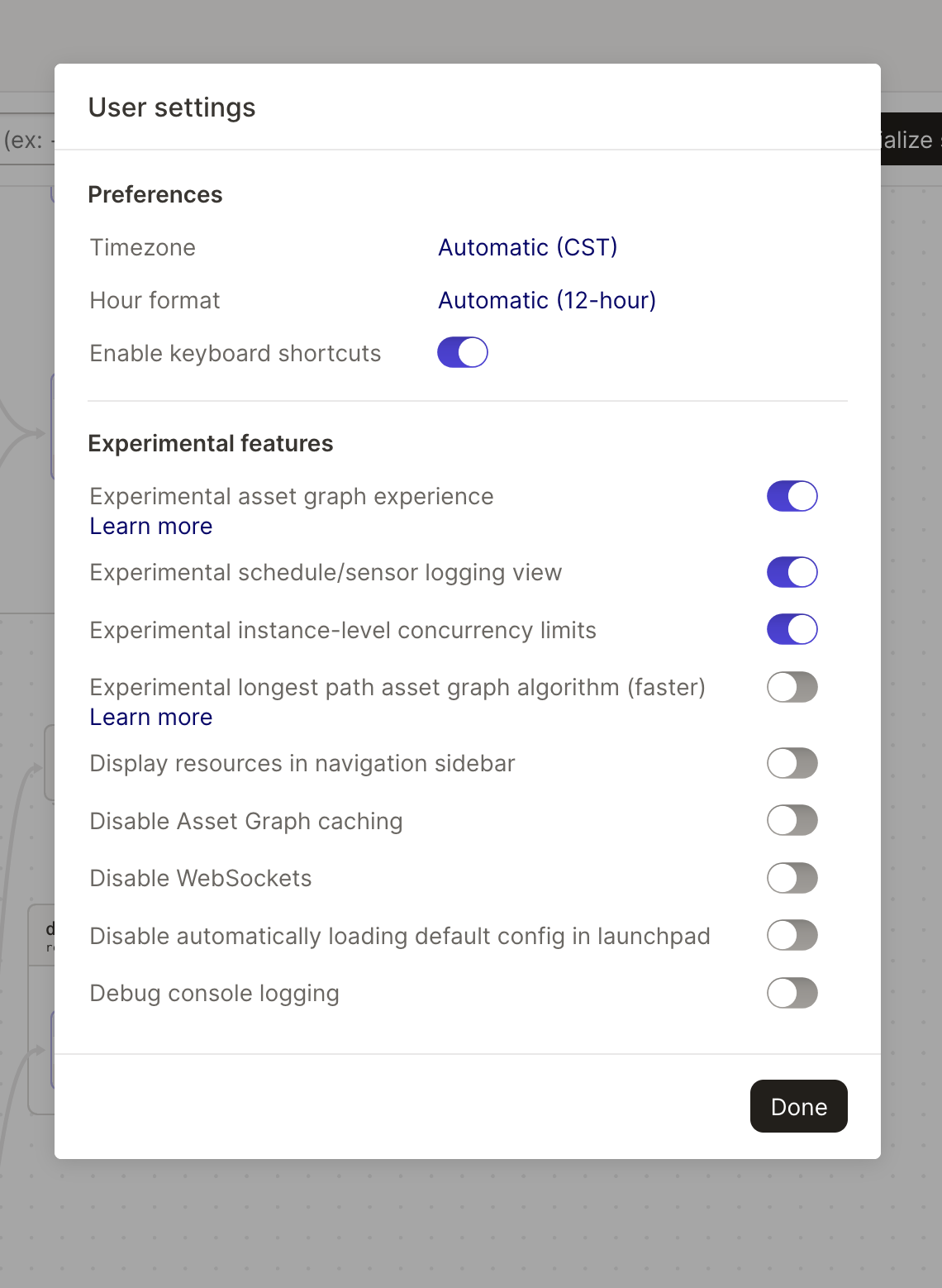The image depicts a user settings menu overlaid on a grey background screen. The pop-up menu has a white background. In the upper left corner, "User Settings" is displayed in black text, followed by a thin grey line that runs horizontally across the menu.

Below the heading, the menu is structured as follows:

1. **Preferences Section:**
   - **Time Zone:** On the right, it shows "Automatic (CST)" in blue text.
   - **Hour Format:** Displays "Automatic (72 hour)" in blue text to the right.
   - **Enable Keyboard Shortcuts:** This option includes a toggle. The toggle background is dark cobalt blue, and the circular switch is white and positioned to indicate it is on.

2. **Experimental Features Section:**
   - A faint grey line separates this section from the one above.
   - **Experimental Asset Graph Experience:** Accompanied by a "Learn more" link in blue text, it is toggled on.
   - **Experimental Schedule/Sensor Logging View:** This is toggled on.
   - **Experimental Instance Level Concurrency Limits:** Also toggled on.
   - **Experimental Longest Path Assist Graph Algorithm Faster:** Includes a "Learn more" link in blue text, this feature is toggled off.
   - **Display Resources in Navigation Sidebar:** Toggled off.
   - **Disable Asset Graph Caching:** Toggled off.
   - **Disable Web Sockets:** Toggled off.
   - **Disable Automatically Loading Default Config in Launchpad:** Toggled off.
   - **Debug Console Logging:** Toggled off.

At the bottom right of the menu, there is a black rectangle with rounded corners containing the word "Done" in white text.